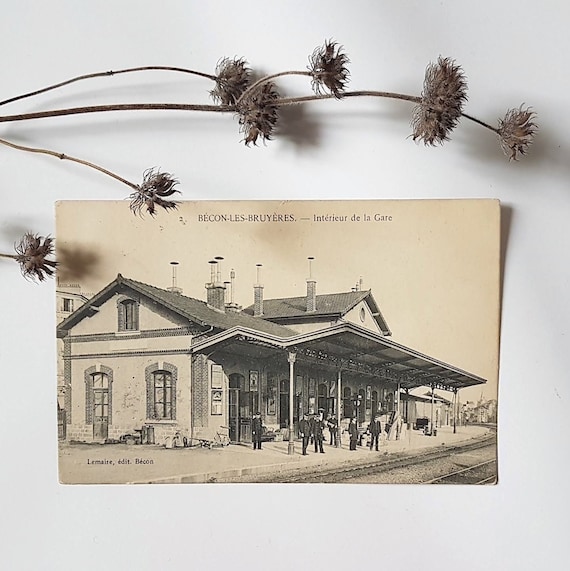The photograph, an old black-and-white postcard with a yellowed, tea-stained background, captures an intricately detailed Victorian-style railway station. The station features a sloping roof and shading projections for waiting passengers. The building's architectural beauty is highlighted by its arch windows. In the lower right corner of the image, railroad tracks extend, grounding the historic scene. People in period attire, likely railway men and passengers, stand outside, engaged in their daily routines. 

Across the beige paper at the top of the image, the text reads “Bécon-les-Bruyères” and “Intérieur de la Gare,” suggesting a French location. In the lower left-hand corner, partly obscured text appears to include the signature "Lemaire, Bécon."

Adding an artistic element, the postcard is carefully placed on a light gray table within a modern white-walled indoor setting. Draped horizontally above the postcard is a dried plant stem, adorned with furry, gray flowers, casting delicate shadows. The combination of the historical image with the natural, textured sprig creates a unique and vintage-inspired wall art piece.